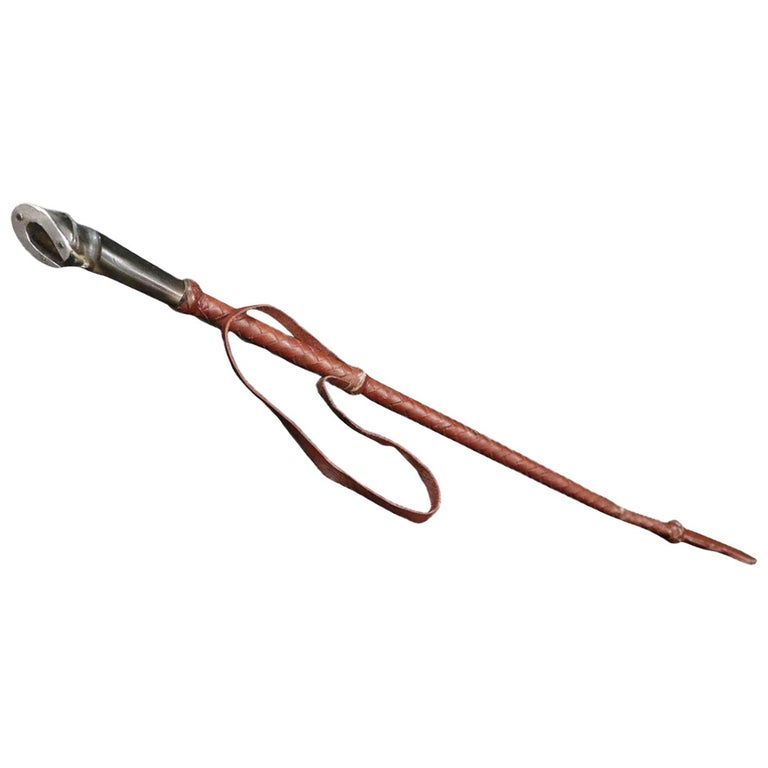The image depicts a large, brown wooden stick set against a completely white background. The stick appears to function as a walking cane and has a knot located towards the middle, giving it a rustic look. It features a leather strap attached around the midpoint, with part of the strap hanging down. The upper portion of the stick is adorned with shiny silver metal, resembling a handle shaped like a horseshoe with two black dots, potentially mimicking bolts. This metal section forms the top of the handle, enhancing the stick's aesthetic appeal. The object extends diagonally from the bottom right side to the top left side. Overall, it's a detailed and prominently displayed walking cane or possibly a historic ornamental staff.